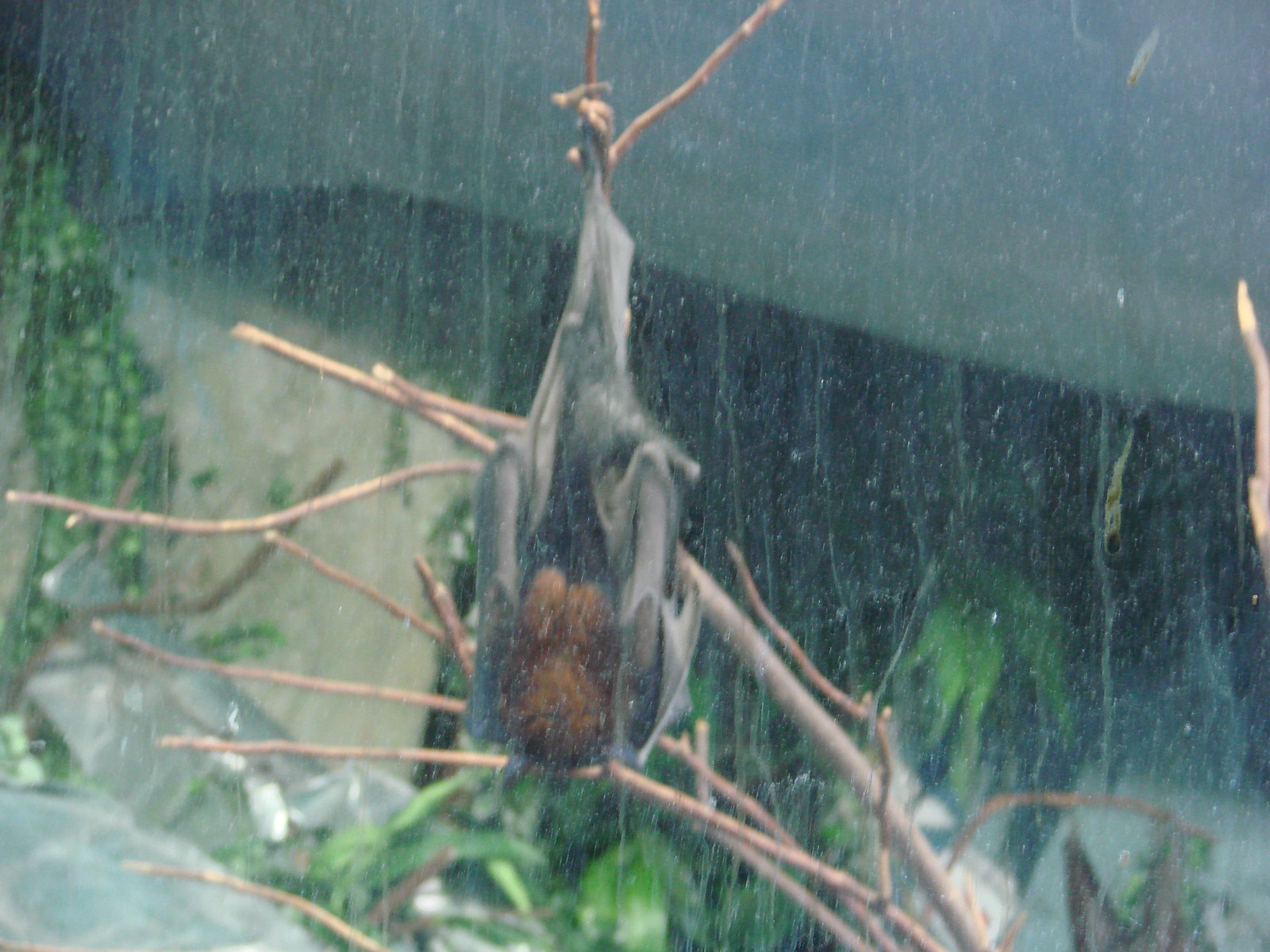A photograph taken through a smudged and water-streaked window, revealing an obscured scene outside. The glass is dirty, with numerous smear marks and dried water spots impeding clear visibility. In the center of the image, somewhat out of focus, a large bat hangs upside down from a thin, leafless branch. The bat's light brown, furry head is visible, while its gray wings are folded close to its body. Surrounding the bat, there's a mix of green foliage and additional branches. In the background, partially concealed by the grimy window and reflected light, are more trees and a structure resembling a green canopy above a dark area, possibly a cement rock wall with a cave-like indentation. This photograph captures the bat in daylight, providing an interesting juxtaposition of the indoor and outdoor environments.